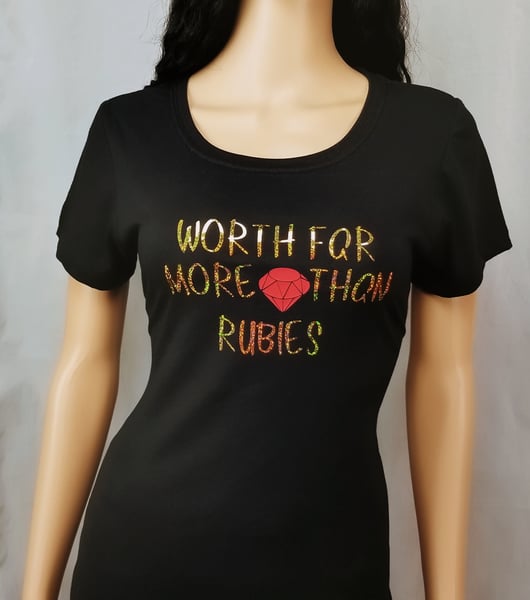In the photograph, a light-skinned woman, or possibly a mannequin, is showcased against a simple white background. She is wearing a fitted, short-sleeve dark brown t-shirt with a scooped neckline. The focus is on the t-shirt, which bears the phrase "WORTH FAR MORE THAN RUBIES" in gold capital letters. Centrally placed between the words "MORE" and "THAN" is a graphic of a pink ruby gem. The text is distributed over three lines: "WORTH FAR" on the first line, "MORE" and the pink ruby icon on the second, and "THAN RUBIES" on the third. The woman is shown from the neck down to just above the wrists, with dark curly hair visible at the top of the image. Her skin appears glossy, suggesting she might be covered in oil or it could be a reflection, implying the figure might be a mannequin. Her arms are relaxed by her sides, focusing the attention on the detailed message of her t-shirt.